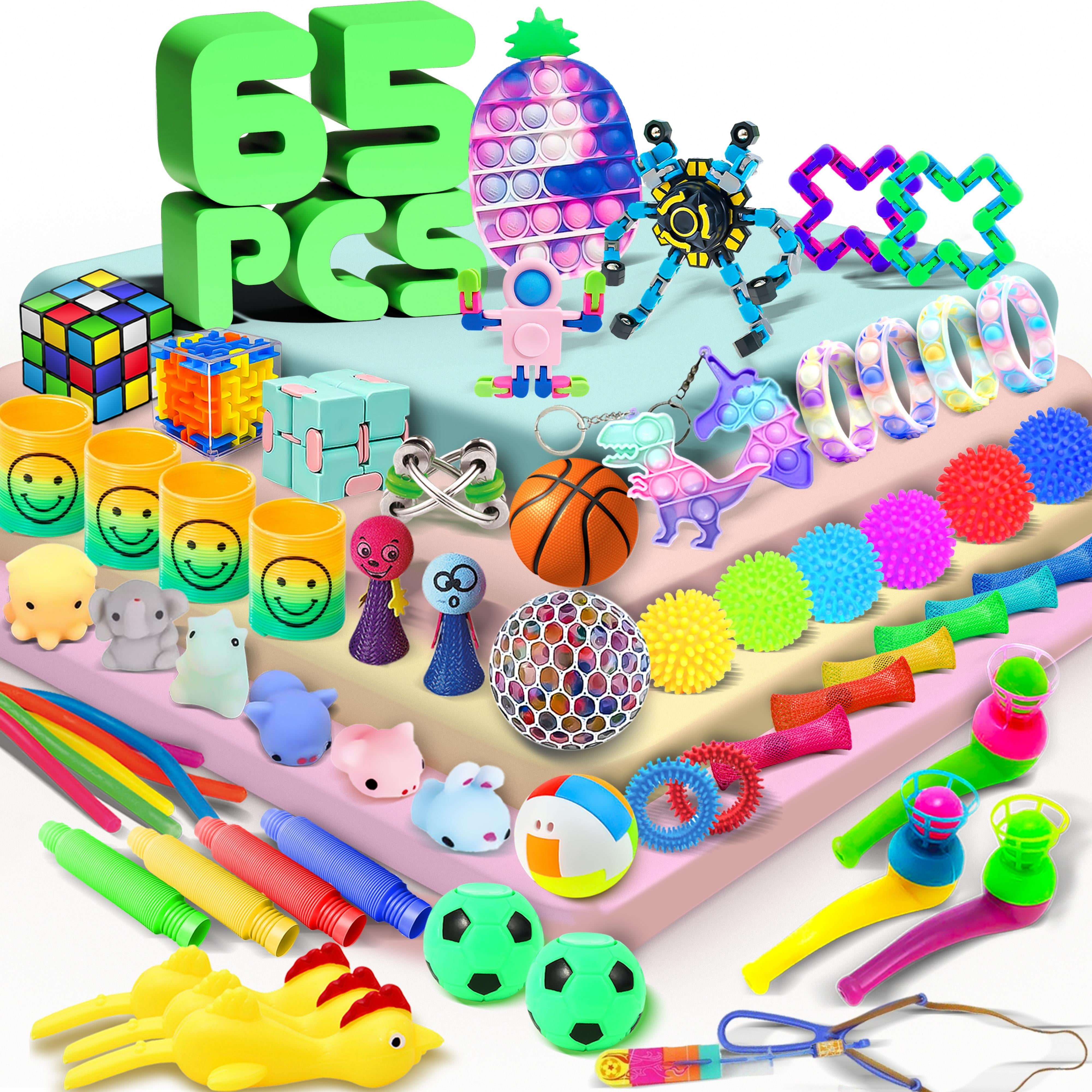This image displays a 65-piece set of toys meticulously arranged on a multi-tiered, pyramid-style platform with a base that narrows as it ascends. At the top of the image, vibrant green block lettering announces "65 pieces." Among the colorful collection, prominent items include a trio of pop fidget toys shaped like a pineapple, dinosaur, and unicorn in hues of pink, blue, and purple. The tiers host an array of additional toys, including a Rubik's Cube, a basketball, and two green soccer balls. Other items include Chinese finger traps, koosh balls, squishy objects, and various animals. The collection also features three rubber chickens, a disco ball, bendable robots, plastic Xs, children's games, cups resembling slinkies, and an assortment of balls and bracelets, all meticulously placed along the edges of the tiered platform.